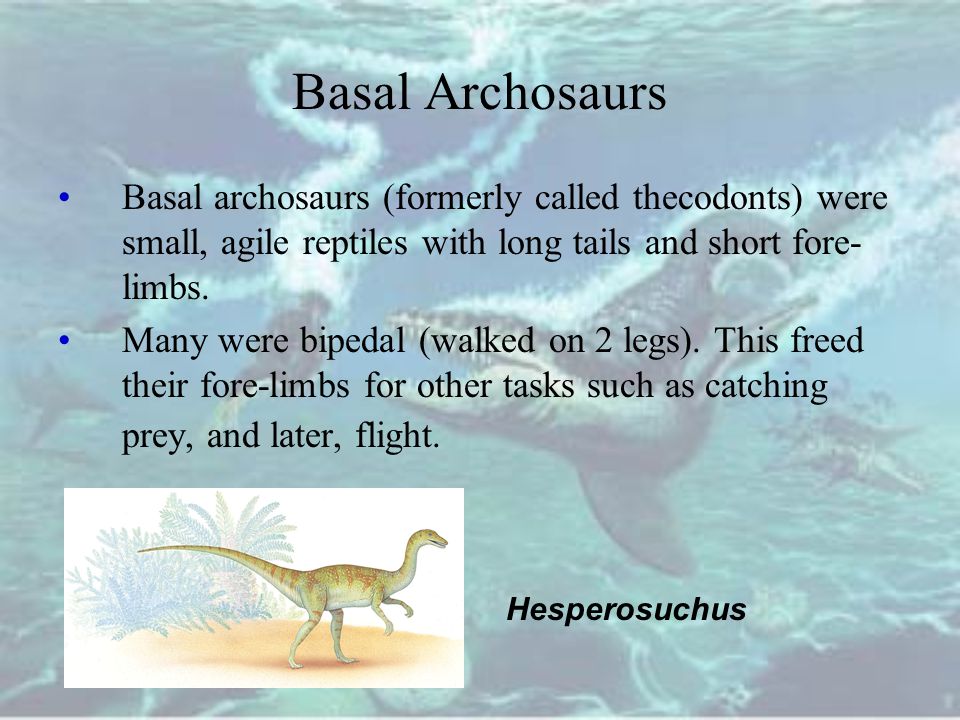The image features an underwater scene with several sea creatures actively swimming, leaving trails of white bubbles in their wake. Superimposed on this background is text in black Times New Roman font, centered at the top, reading "Basal Archosaurs." Below the title are two blue bullet points, also in Times New Roman font. The first bullet point states, "Basal archosaurs, formerly called thecodonts, were small agile reptiles with long tails and short forelimbs." The second bullet point adds, "Many were bipedal and walked on two legs. This freed their forelimbs for other tasks such as catching prey and later flight." In the bottom left corner, there's a small image depicting Hesperosuchus, a yellow and orange dinosaur standing on its hind legs, with a long neck and tail, facing right. Background foliage is faintly visible behind its tail.